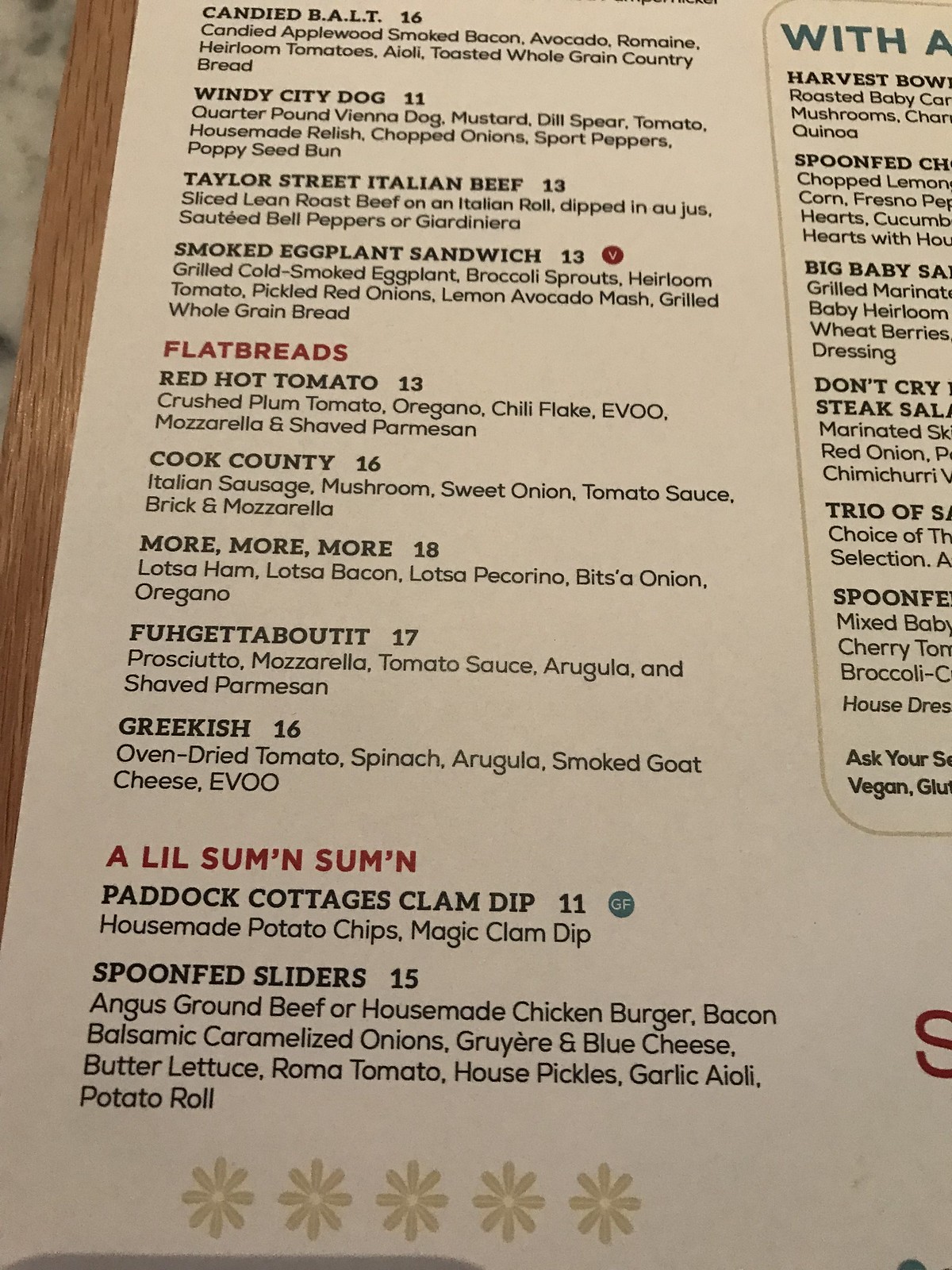**Detailed Caption:**

The photograph showcases a detailed menu framed in wood or possibly leaning against a wooden surface, with a glimpse of the background in the upper left corner. The menu is printed on cream-colored, sturdy paper stock and lists a variety of mouth-watering dishes. 

**Sandwiches:**
1. **Candied B.A.L.T. $16**
   - Candied applewood smoked bacon
   - Avocado
   - Romaine lettuce
   - Heirloom tomatoes
   - Aioli
   - Toasted whole grain country bread

2. **Windy City Dog $11**
   - Quarter-pound Vienna dog
   - Mustard
   - Dill pickle spear
   - Tomato
   - House-made relish
   - Chopped onion
   - Sports peppers
   - Poppy seed bun

3. **Taylor Street Italian Beef $13**
   - Sliced lean roast beef on an Italian roll
   - Dipped in au jus
   - Sauteed bell peppers or giardiniera

4. **Smoked Eggplant Sandwich $13** (Vegan)
   - Grilled cold smoked eggplant
   - Broccoli sprouts
   - Heirloom tomato
   - Pickled red onions
   - Lemon avocado mash
   - Grilled whole grain bread

**Flatbreads:**
1. **Red Hot Tomato $13**
   - Crushed plum tomato
   - Oregano
   - Chili flake
   - Extra virgin olive oil (E.V.O.O)
   - Mozzarella
   - Shaved parmesan

2. **Cook County $16**
   - Italian sausage
   - Mushroom
   - Sweet onion
   - Tomato sauce
   - Brick and mozzarella

3. **More, More, More $18**
   - Lots of ham
   - Lots of bacon
   - Lots of pecorino
   - Bits of onion
   - Oregano

4. **Forget About It $17**
   - Prosciutto
   - Mozzarella
   - Tomato sauce
   - Arugula
   - Shaved parmesan

5. **Greek-ish $16**
   - Oven-dried tomatoes
   - Spinach
   - Arugula
   - Smoked goat cheese
   - E.V.O.O

**A Little Something Something:**
1. **Paddock Cottages' Clam Dip $11** (Gluten-Free)
   - House-made potato chips
   - Magic clam dip

2. **Spoon-Fed Sliders $15**
   - Angus ground beef or house-made chicken burger
   - Bacon balsamic
   - Caramelized onions
   - Gruyere and blue cheese
   - Butter lettuce
   - Roma tomato
   - House pickles
   - Garlic aioli
   - Potato roll

Set against a wooden backdrop, this menu offers a delectable selection of sandwiches, flatbreads, appetizers, and sliders, each described with intricate detail to entice any food lover.